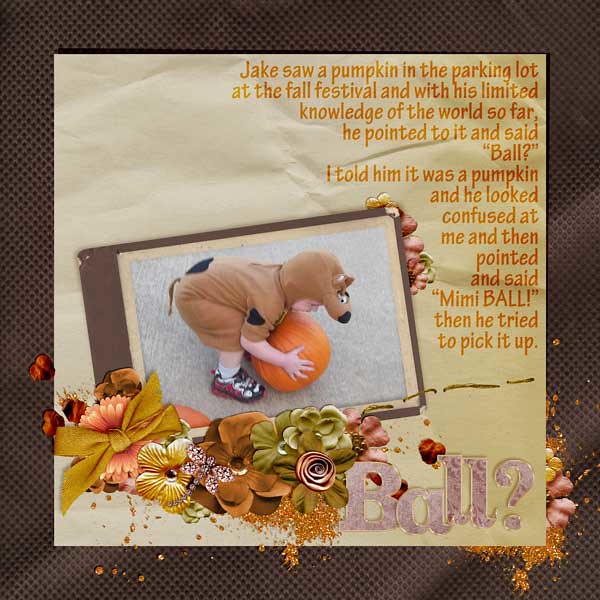The image is that of a decorated scrapbook page featuring a photograph of a little Caucasian boy with white skin. The boy, dressed in a Scooby-Doo Halloween costume, is captured in the moment as he bends over and tries to pick up a large, spherical orange pumpkin in the parking lot at a fall festival. In the background, the scrapbook page is adorned with floral decorations and glitter, adding to the festive, autumnal feel. The photograph also includes text in orange that narrates the story: "Jake saw a pumpkin in the parking lot at the Fall Festival, and with his limited knowledge of the world so far, he pointed to it and said, 'ball'. I told him it was a pumpkin, and he looked confused at me and then pointed and said 'meanie ball'. Then he tried to pick it up." At the bottom right corner of the page, "ball?" is written in goldish letters, accentuating the child's adorable confusion. The entire presentation gives off a modern and heartfelt vibe, capturing a precious memory likely cherished by a family member.